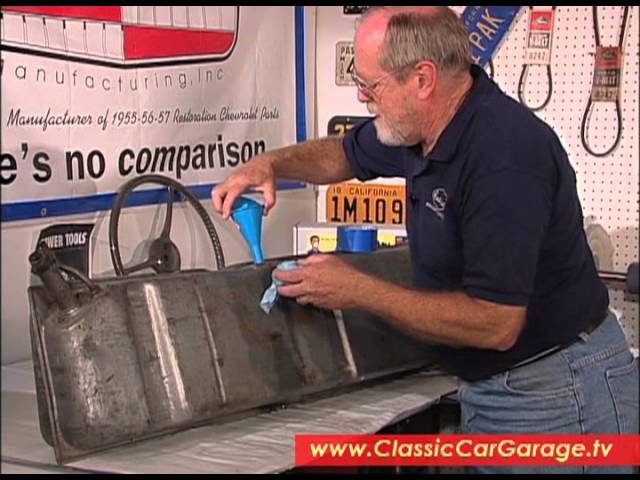The image appears to be a screenshot from a TV show, evident from the yellow text on a red background at the bottom that reads "www.classiccargarage.tv." The setting is a classic car workshop filled with nostalgic elements such as posters and vintage license plates adorning the walls, as well as fan belts hung on a pegboard. 

Prominently featured in the image is an older, bald man with a neatly trimmed gray beard and glasses. He is wearing a dark blue polo shirt and light blue jeans. The man is diligently working at a workbench, focusing on a large, silver, horizontal container that seems to be a car's fuel tank. He holds a light blue funnel over an opening in the tank with his right hand, while his left hand grips a blue rag. One notable poster in the background reads, "There's No Comparison, Manufacturing of 1955-56-57 Rubitoid Chevrolet Parts." This detailed scene captures the essence of a vintage car restoration shop.